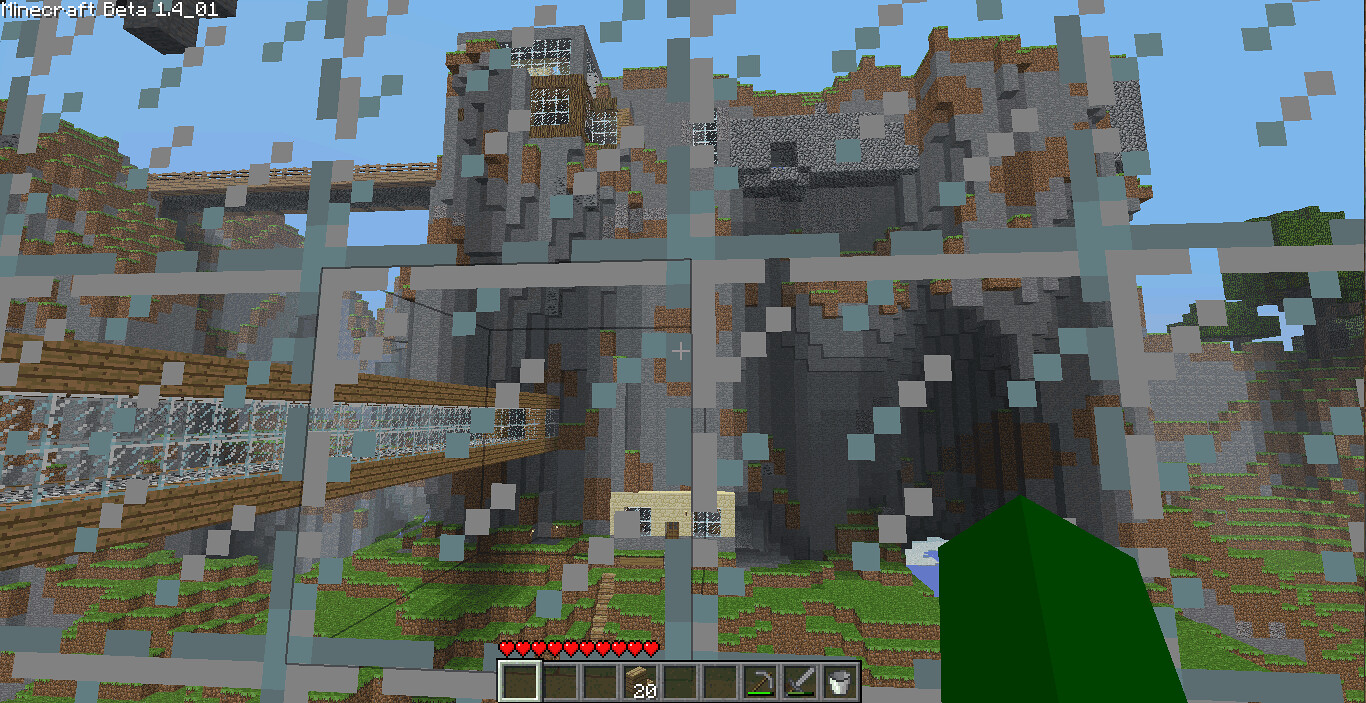In this detailed screen capture from Minecraft Beta 1.4-01, a first-person perspective reveals the classic blocky, pixelated landscape characteristic of the game. The player's view is framed by the green rectangular hand typically holding a weapon, possibly a sword. The health bar, represented by red hearts, and the inventory bar populate the bottom left corner, containing various items that are indiscernible. The scene is dominated by a wall constructed of pixelated glass blocks, detailed with gray and blue highlights to emphasize their texture.

Beyond the glass wall lies a sprawling outdoor environment. A vibrant, green grassy terrain extends outward, interspersed with various blocky formations indicative of Minecraft's procedural generation engine. In the distance, a structure resembling a fortress composed of concrete or stone blocks appears, connected by what seems to be an elevated walkway or bridge. The fortress stands against a backdrop of a bright blue sky, typical of Minecraft’s clear weather. The overall aesthetic retains a low-resolution, cartoon-like charm, with occasional pixel artifacts that might appear as missing squares within the image.

This scene encapsulates the quintessential elements of Minecraft's visual style, showcasing its iconic block-based world and the early beta stage nuances.